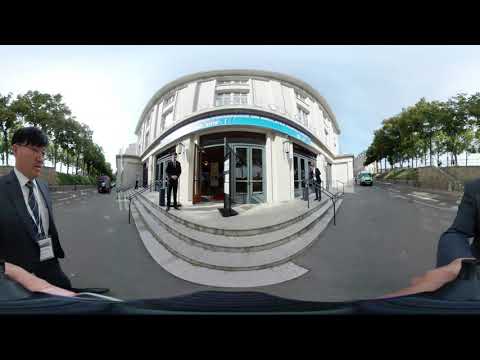The image captures a detailed scene in front of a two-story white building, rendered with a fisheye lens giving it a slightly distorted, wide-angle view. The main focus is the entrance, which features outward-opening double doors at the top of three wide, white steps. Standing on the left is a man with glasses, dressed in a black business suit with a black and white striped tie, and a white ID card hanging from a lanyard. Another person in a gray suit with a patterned tie is seen standing near the doorway. To the right of the door, a third man in a coat appears to be entering another door. The building has a distinctive blue border running between its two stories. The surrounding scene includes roads on both sides with some vehicles and rows of tall green trees lining the sidewalks. The sky above is mostly blue with some white hues, and the sun is positioned towards the left of the image, emphasizing the natural light in the scene.